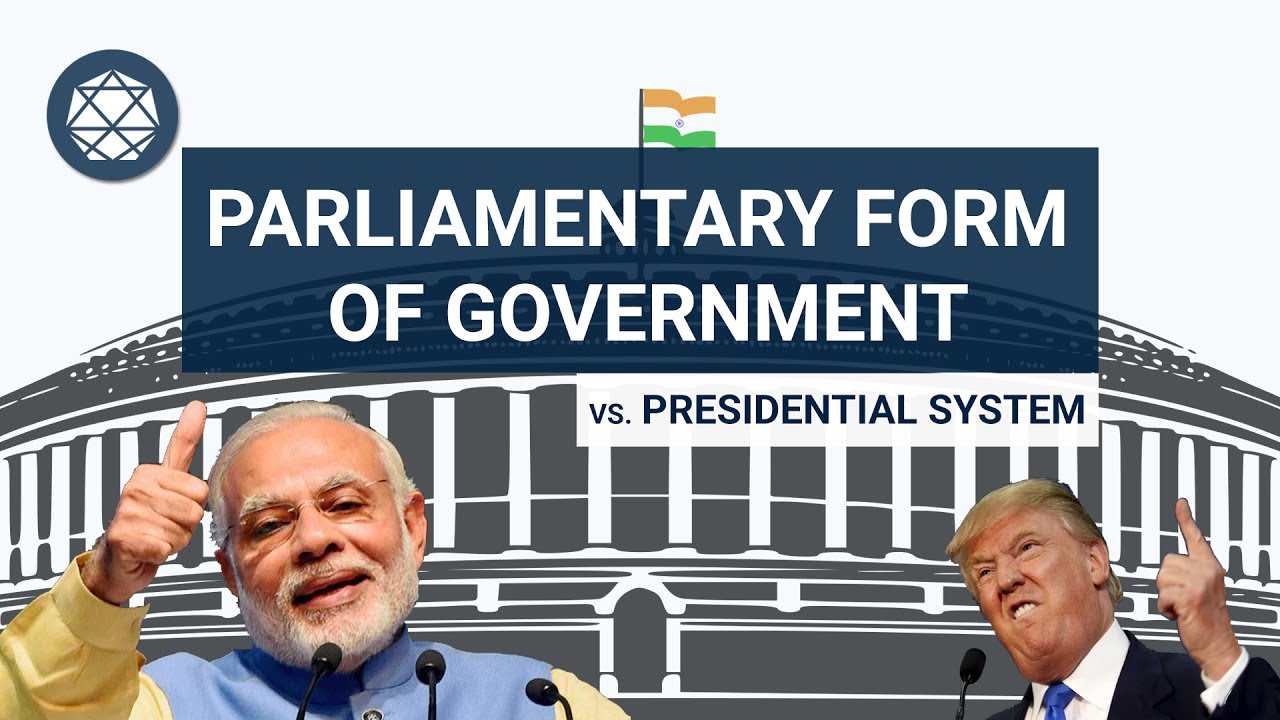The meme features an all-white background with a blue and white star encircled by a thick blue ring in the upper left-hand corner. At the top of the image, just above a central blue rectangle, there is a flag that appears to be of a Middle Eastern or possibly Indian origin, set against what looks like the clip art of a blue and white round building, resembling a government-style structure. 

Inside the blue rectangle, the words "PARLIAMENTARY FORM OF GOVERNMENT" are displayed prominently in white, uppercase letters. Below this is a smaller white rectangle containing the words "VERSUS PRESIDENTIAL SYSTEM" in all capital letters, in blue font.

To the left of the lower half, beneath the blue rectangle, stands an older man, possibly a political leader from Turkey, the Middle East, or India. He has white hair and a beard, wears glasses, and is dressed in a blue and gold tunic. He is positioned in front of three microphones and is giving a thumbs up.

On the lower right-hand side, under the white rectangle, is a photo of President Donald Trump. He is wearing a black suit with a blue tie and has an angry expression on his face, raising his index finger in a pointing gesture. He stands next to a single microphone.